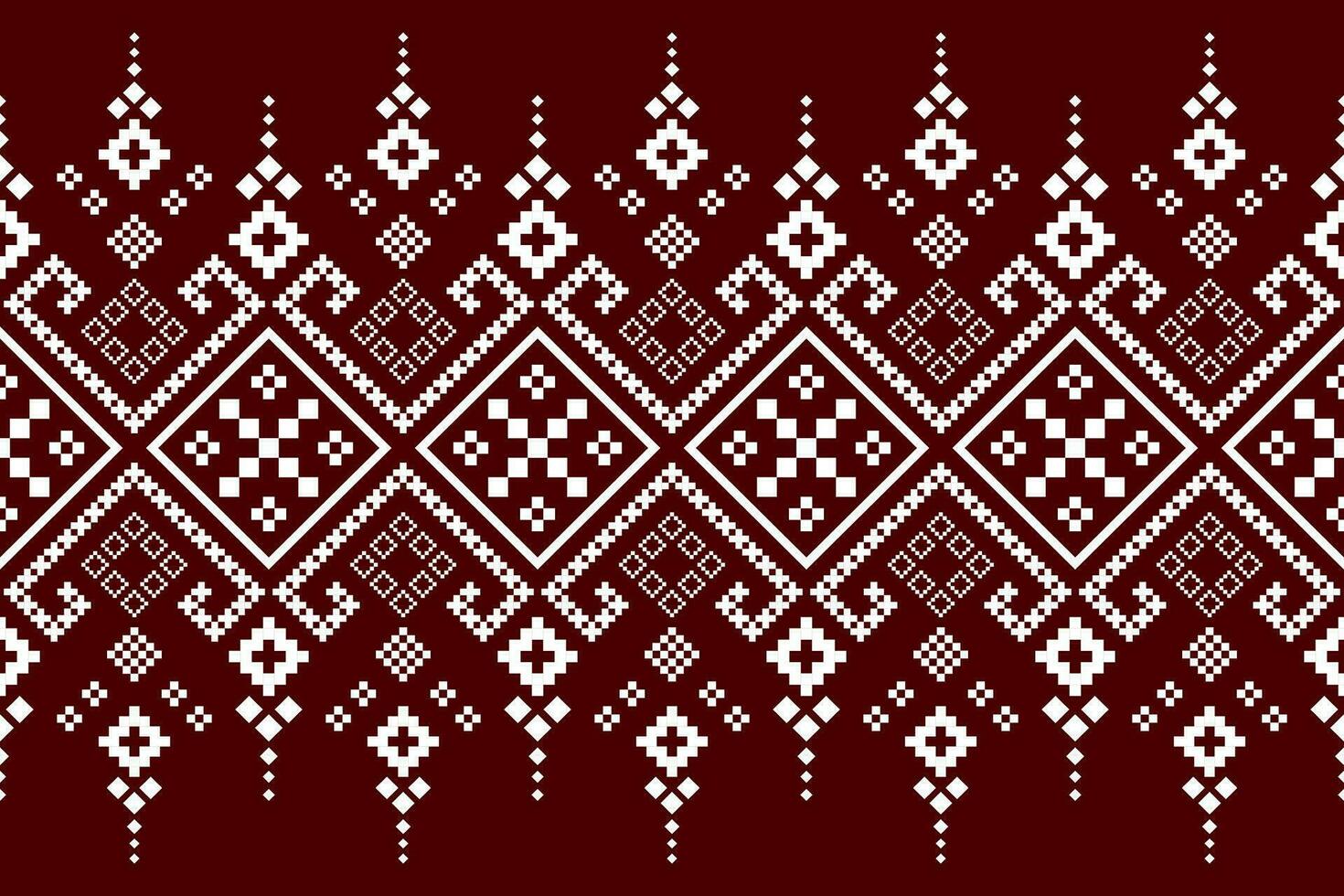The image depicts a complex, quilt-like pattern featuring intricate geometric symbolism from an unknown culture. The backdrop is a deep burgundy, wine-red color, which contrasts sharply with the white designs that dominate the center. The main pattern comprises a series of interconnected, symmetrical squares tilted at 45-degree angles, giving them a diamond-like appearance. Inside each square is an 'X' with a small circle at each intersection, contributing to a sense of dimensionality.

Further contributing to the intricate design, each square is flanked by smaller surrounding squares, lending an impression of larger compositional blocks forming an overall harmonious design. The pattern repeats in a grid-like arrangement across the image. At the top of each diamond shape, there are crown-like, steeple designs that enhance the overall visual complexity. The layout of the design evokes imagery of flowers, crosses, and other geometric shapes through its meticulous arrangement of straight lines and angles.

The symmetry and repetition in the pattern could be reminiscent of traditional quilt designs, though the rich burgundy and precise geometric elements lend it an air of cultural symbolism that is both intricate and captivating.